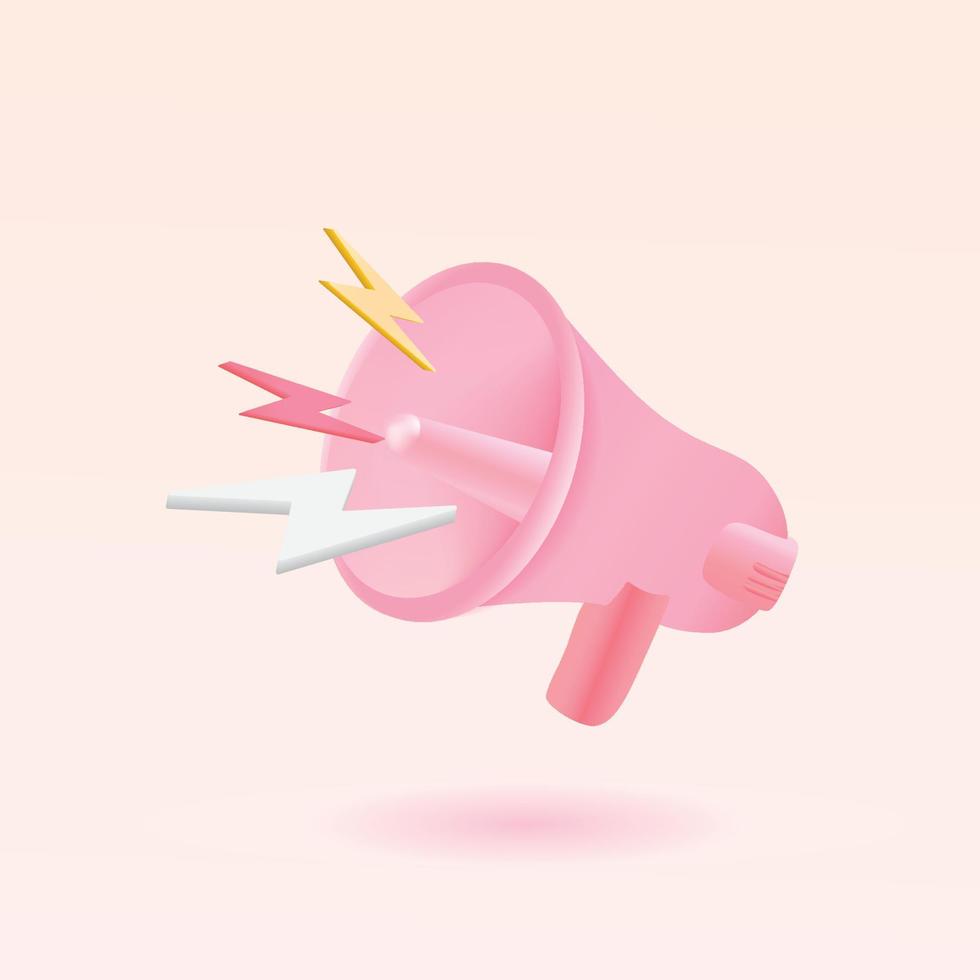The image features a detailed, graphic design illustration of a floating pink megaphone against a light peach background with subtle shadowing underneath. The megaphone, which has a darker pink handle, is depicted in a 3D, vector art style, giving it a cartoony yet realistic appearance. On the side of the megaphone, there's a pink dial with three notches, and a small protruding device resembling a microphone attachment. In the middle of the megaphone, a spoke is visible. Radiating from the megaphone’s opening are three lightning bolt shapes that symbolize sound: the smallest bolt at the top is yellow with a slightly darker yellow shadow, the middle bolt is dark pink matching the handle's shade, and the largest and bottom bolt is white with a gray drop shadow. The megaphone is oriented to the left, and the background features a slight shadow beneath it, emphasizing its floating appearance.